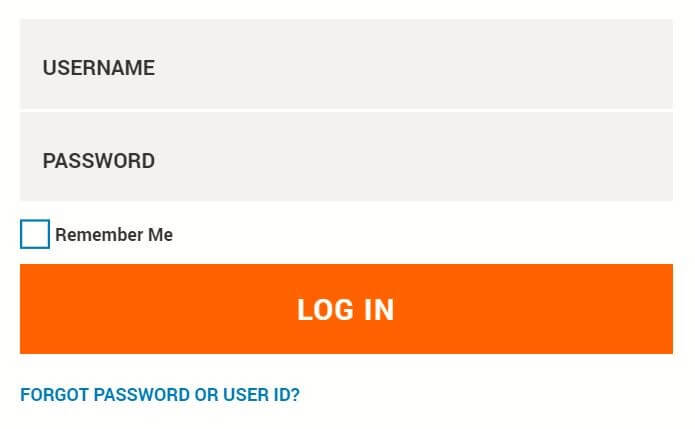A screenshot of a basic login page for a website featuring two primary input fields is displayed. The first input field is labeled "Username" and remains empty, inviting the user to type in their credentials. Directly below, the second field, similarly unpopulated, is labeled "Password." Beneath these fields, there is a checkbox option accompanied by the label "Remember me," allowing users to enable their browser to store their login information for future visits. This helps in bypassing the need for re-entering credentials on subsequent visits. Below the checkbox, a large, prominent orange button labeled "Login" stands out, ready to be clicked once the necessary information has been filled in. At the very bottom of the screenshot, a link reads "Forgot Password or User ID," providing an accessible option for users who may need to recover their login details. Despite the uniformity and simplicity of this typical login page, no further information is available to identify the specific website it belongs to.